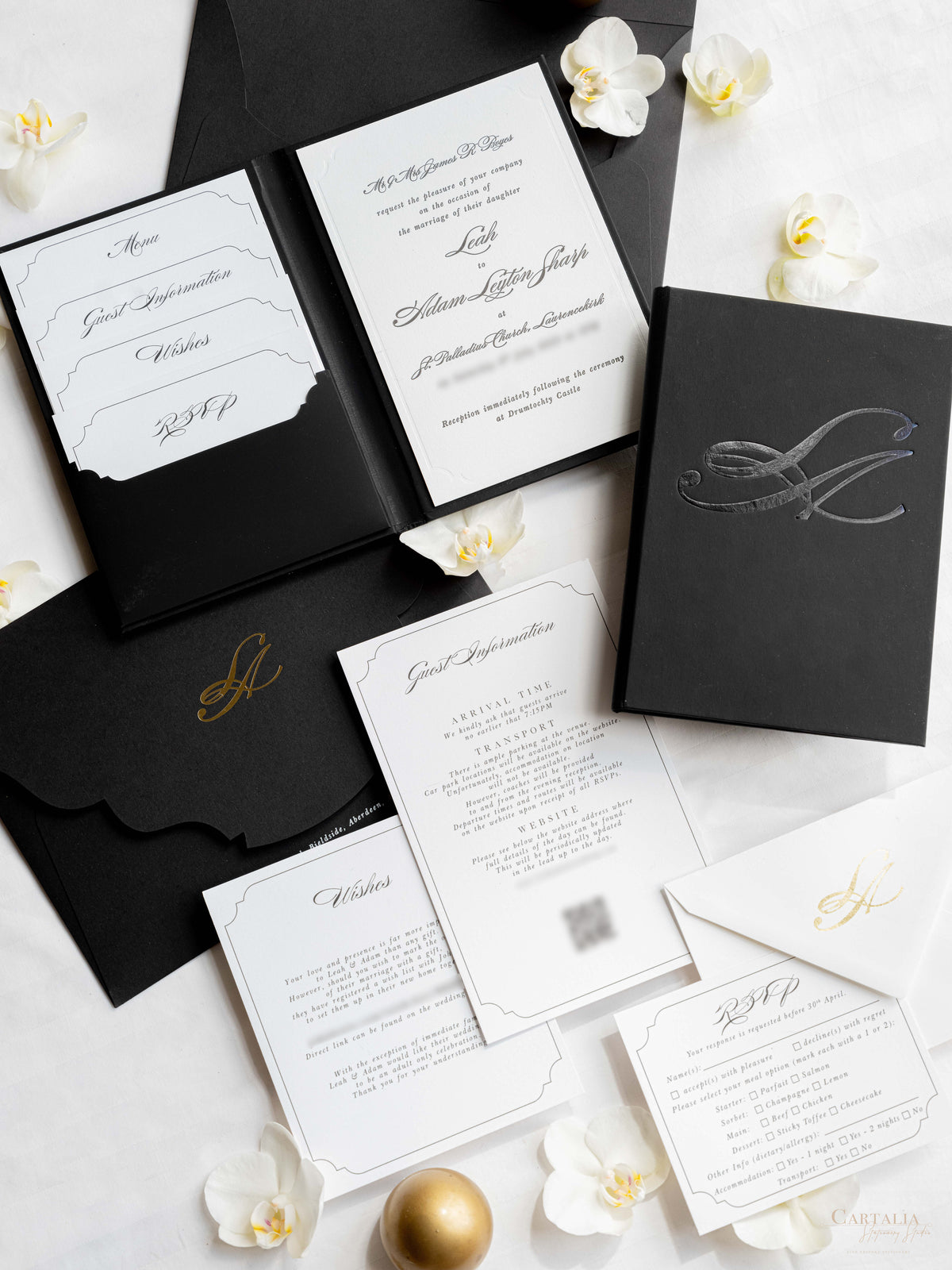This vertical image, predominantly in black and white, functions as an intricate advertisement for a wedding invitation set. The composition features a stark white background with a black envelope prominently placed. Overlaying the envelope is an array of essentials for a polished wedding suite: the menu, guest information, wishes, and RSVP cards. To the right, a visually striking white invitation card is displayed, embellished with elegant, flourish-like calligraphy. Below this, another black envelope features the gilded initials "S.A." in gold.

Additionally, the setup includes what appears to be a book cover in leather with the same initials "S.A." embossed in glossy black against a matte black backdrop. Scattered throughout the scene are various guest invitations, wishes, and RSVP cards. Enhancing the sophistication of the arrangement, white orchids are delicately interspersed, while a gleaming gold ball adds a touch of opulence at the bottom of the image. This meticulous layout on what seems like a black table creates a visually arresting ensemble, capturing the essence of a luxurious wedding invitation suite.